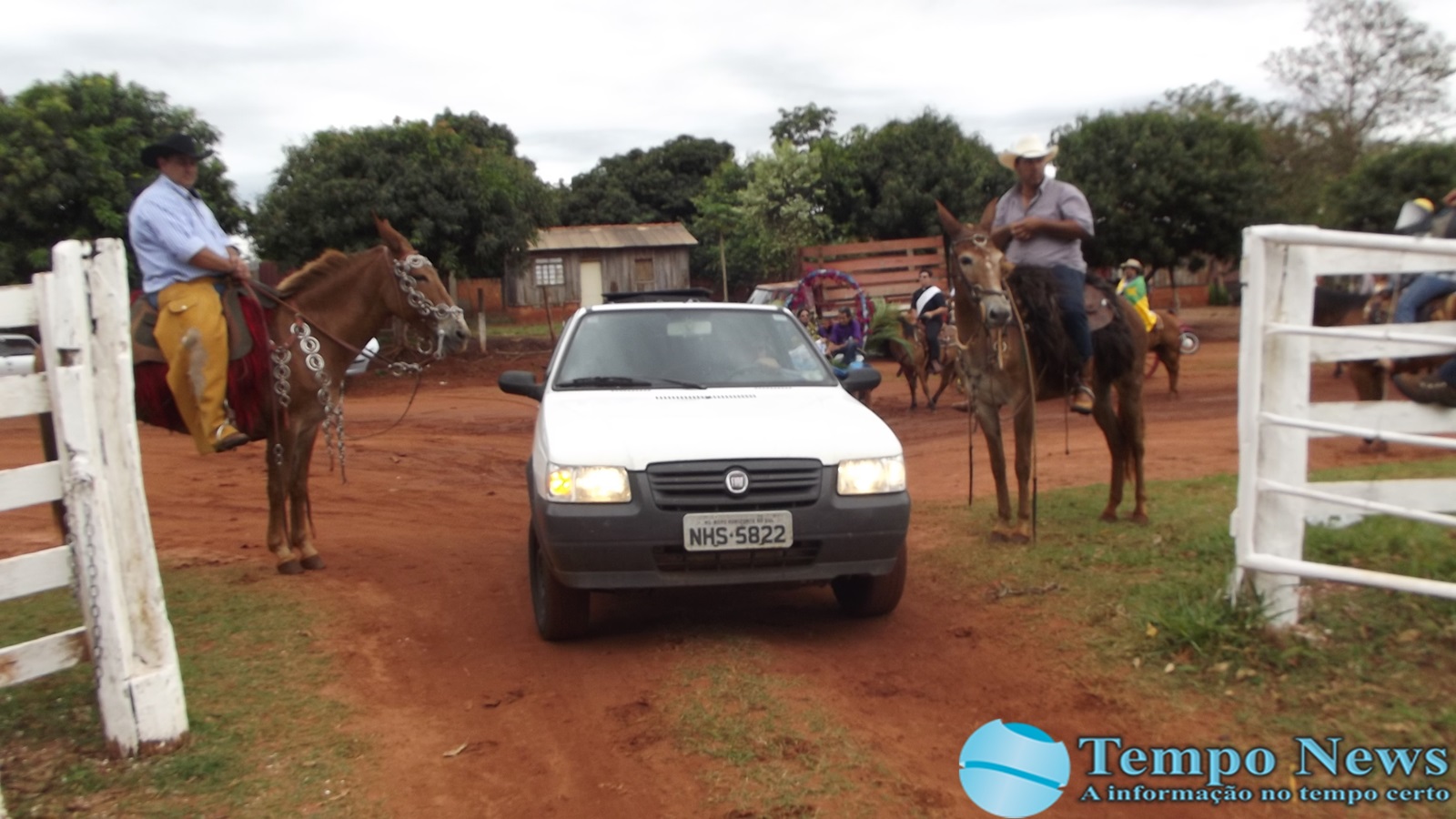In this image, a small white car with the license plate NHS 5822 is positioned centrally on a muddy, dirt-covered area with patches of grass, surrounded by a rural, farm-like setting. To the left and right of the vehicle stand two brown horses, each ridden by men dressed in western attire: the rider on the left wears a blue shirt, yellow trousers, and a black cowboy hat, while the rider on the right sports a grey shirt, navy blue pants, and a white cowboy hat. Another visible horse rider, partially obscured, positions a brown horse behind the white wooden fence on the right. Additional riders can be spotted in the background, including one wearing a black and white shirt and another draped in a green and yellow flag with a yellow logo, while sporting a black cowboy hat. A small wooden building, possibly a hut or barn, stands in the background, accompanied by lush green trees under a heavily clouded sky. There are more vehicles visible behind the central car. The scene is enclosed by white wooden fences and open gates on either side. In the bottom right corner of the image, a blue circular logo with the words "TEMPO NEWS, INFO MAKE COW, NO TEMPO SETTLE" is present.